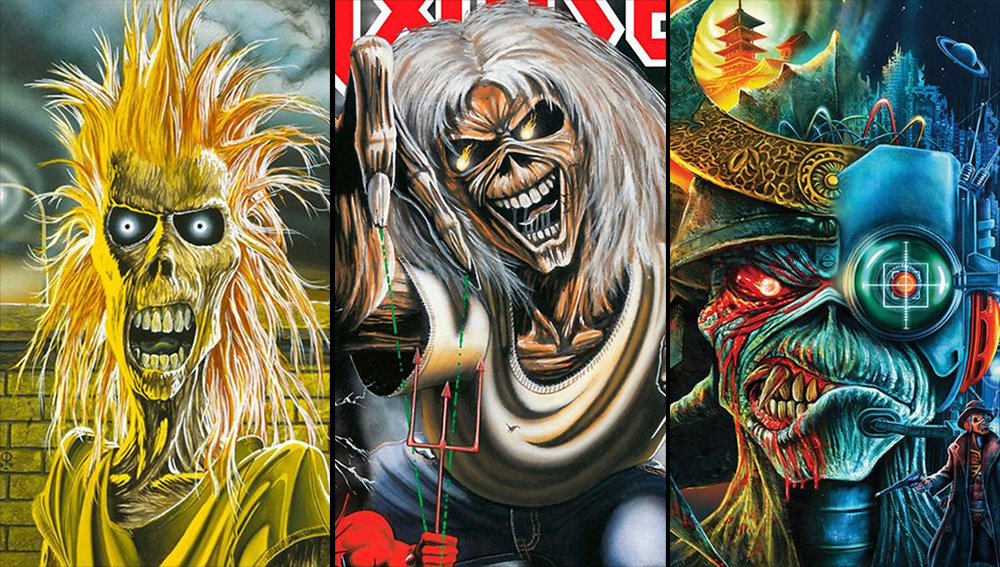The image is a detailed digital artwork poster divided into three vertical sections, each featuring an Iron Maiden-style zombie. 

In the left section, a yellow zombie with spiky long blonde hair and glowing blue eyes snarls fiercely, displaying its giant teeth. It stands against a yellow brick wall, under a dark, gray sky, and wears a yellow shirt. 

The middle section depicts a zombie that resembles an old person with long, white hair and hollow, fiery eyes. It is clad in a white shirt and blue jeans, with a menacing grin on its brown face. At the bottom corner, the top of a devil's head with a pitchfork adds to the eerie atmosphere.

The right section shows a cybernetic zombie with a Viking-like helmet. It has a mechanical eye designed as a digital target, while the left side of its face is grotesquely bloodied. An arrow protrudes from its chin, pointing to the right. A cowboy with a pistol appears in the bottom corner, enhancing the chaotic feel of this dark, dystopian scene.

Each section combines strong, vibrant colors and detailed, grotesque features, epitomizing Iron Maiden's iconic and intense art style.